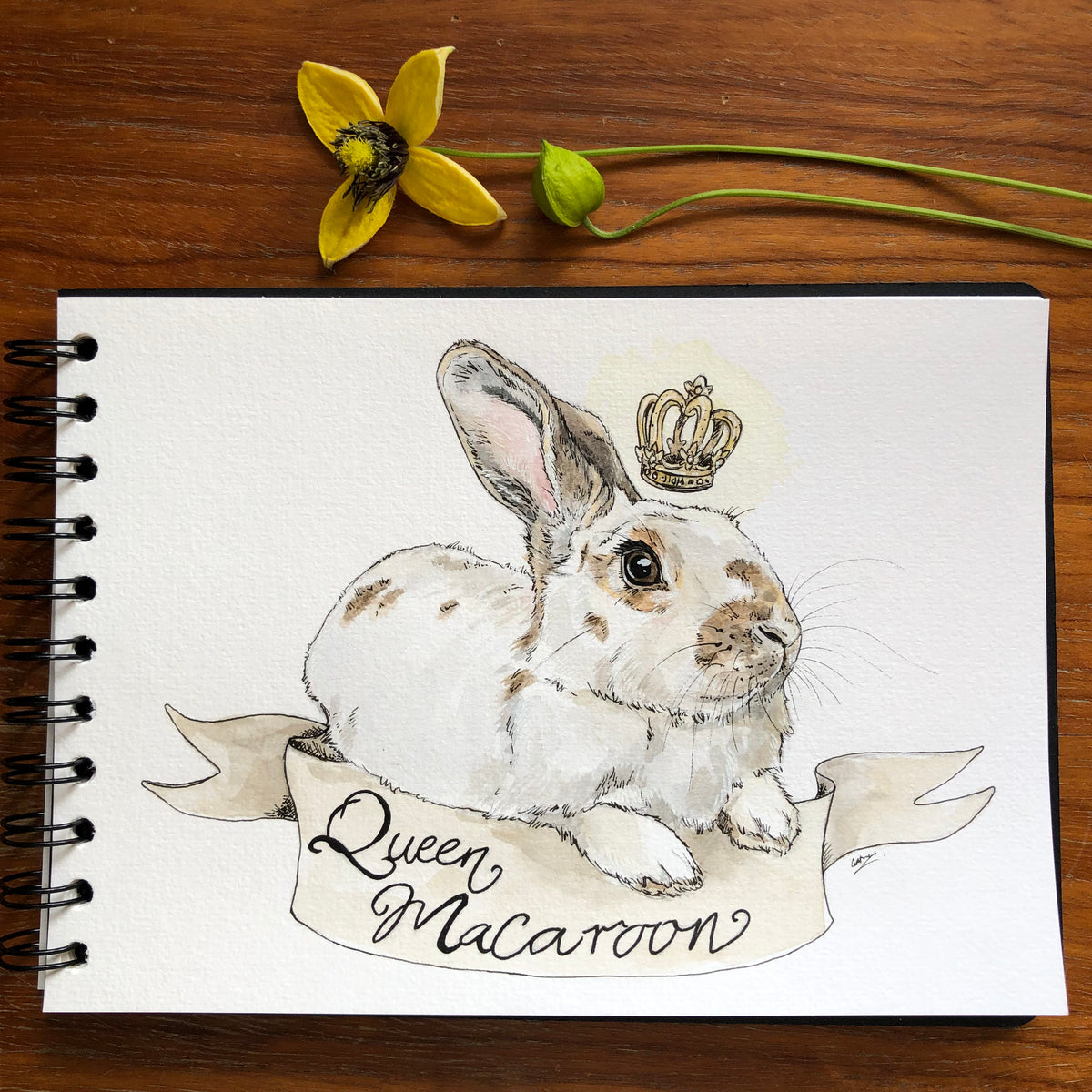The image showcases an artist's spiral-bound sketchbook, oriented with the binding on the left, resting on a light tan wood grain surface. The notebook contains a detailed drawing of a white rabbit accented with brown spots and brown ears. The rabbit is depicted lying on its belly, front paws extending from beneath its chest, and a golden crown hovering above its head. Below the rabbit is a banner adorned with small wings at each end, inscribed with the black cursive text "Queen Macaroon." Positioned above the notebook is a four-petaled yellow flower attached to a green stem, adding a delicate touch to the composition.